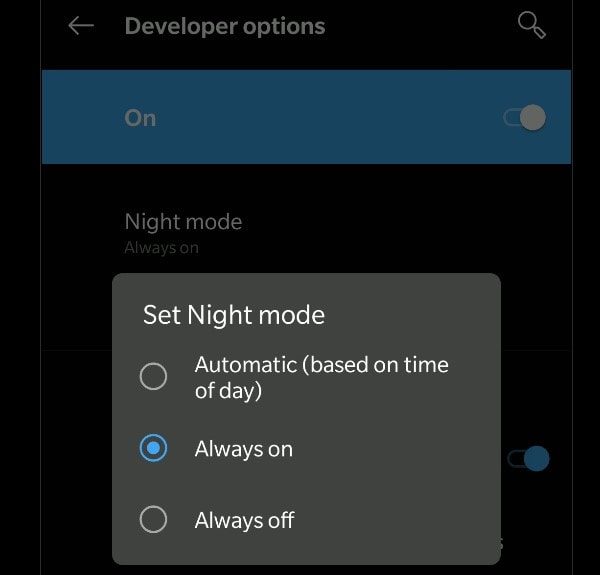The image displays a settings screen from a mobile device, such as a phone or a tablet, featuring a predominantly black background. At the top, in white font, it reads "Developer options," with a left-facing white arrow indicating a back function to return to a previous menu. On the right side of the screen, there is a slanted magnifying glass icon, also in white.

Directly below this, the screen shows a header with a light blue background. On the left side of the header, in bold white letters, it states "ON," and to the right, there is a toggle switch with a white dot positioned to the right, indicating the switch is enabled.

The main section of the screen, continuing with the black background, features the text "Night mode" in white, with smaller gray text beneath it stating "Always on." 

A pop-up window with rounded corners and a medium gray background overlays part of the screen. The heading of the pop-up, "Set night mode," is displayed in larger white font. Below this are three option circles outlined in gray, offering different settings for night mode. The first option reads "Automatic (based on time of day)," the second is "Always on"—which is currently selected, as indicated by its blue outline and a smaller filled-in light blue circle in the center—and the last option is "Always off."

In the background, partially obscured by the pop-up, another toggle switch is visible towards the right side of the screen. This switch is also enabled, indicated by a blue filled-in dot pointed to the right, though the overlay hides the specific setting it controls.